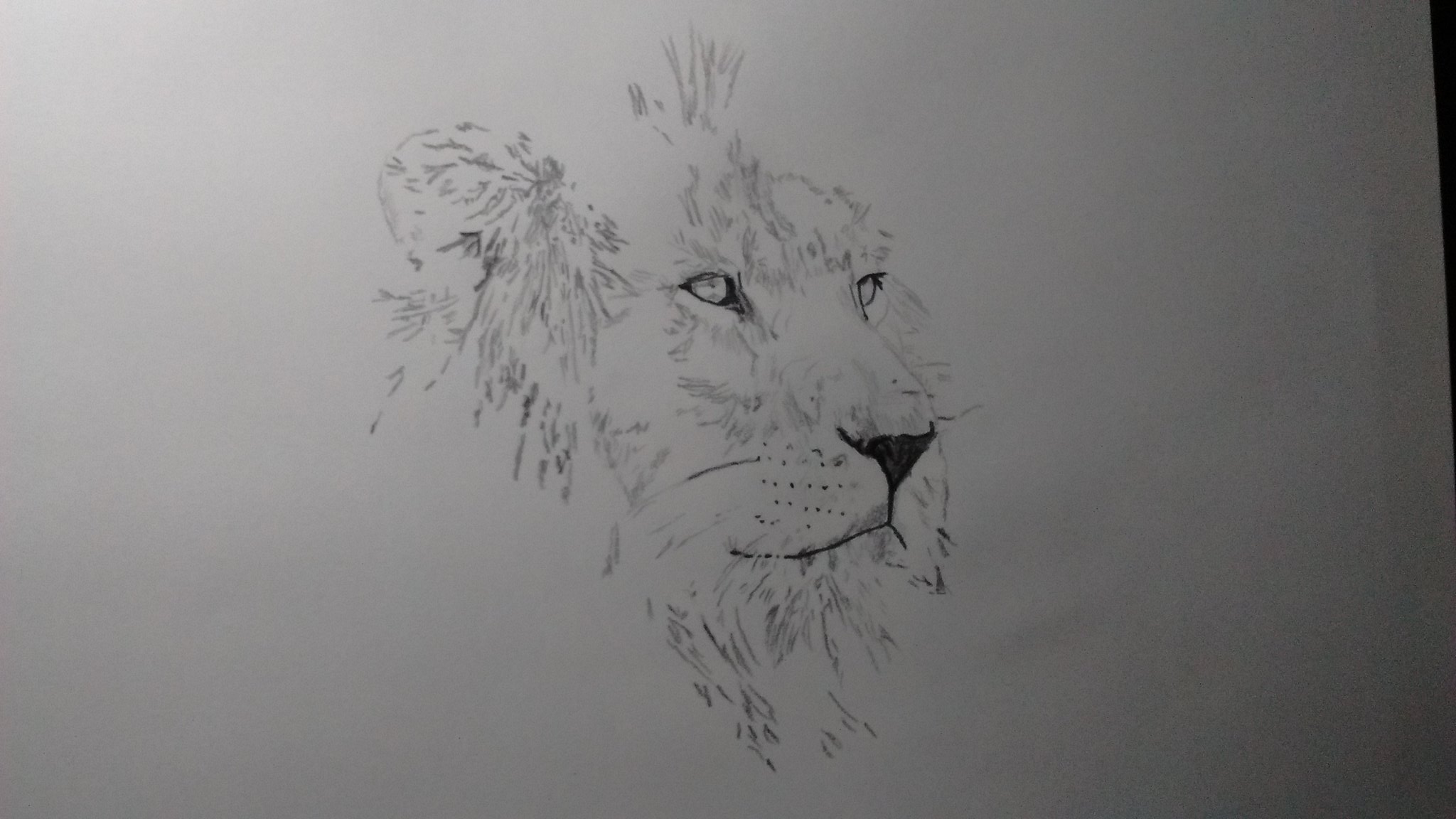This image is a detailed pencil drawing of a lion's head on off-white paper, predominantly viewed from the right side. The lion’s dark, prominent eyes and the distinct nose, which is shaped like an upside-down triangle, draw immediate attention. From the nose, a line extends downward, forming a 'V' shape as it merges with the mouth. The dark grey tone dominates the right side of the drawing, contrasting with the lighter grey shades on the left and upper sections of the paper. The artist has meticulously represented the lion's fur, with bristles rising at the top and the mane flowing downward under the chin towards the neck. One ear is distinctly visible, while the other is obscured. The drawing also includes black lines symbolizing whiskers that emerge from around the nose. Moreover, a sliver of black peeks through from the surface beneath the paper in the upper right-hand corner, adding depth to the image.